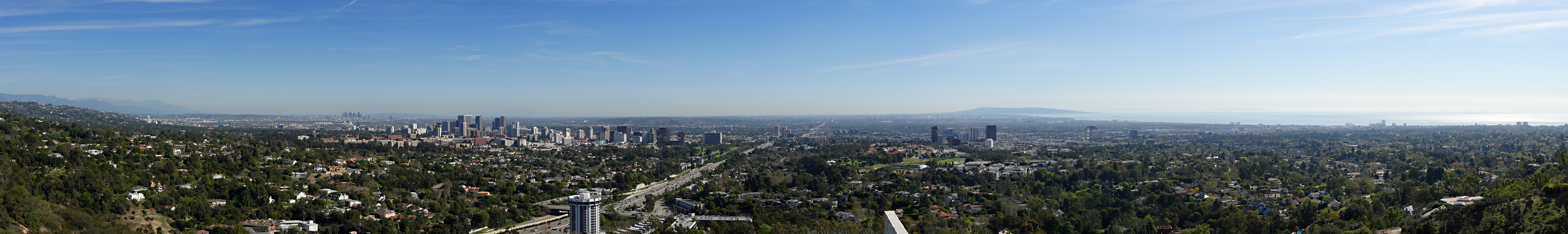This panoramic aerial photograph captures a vast urban sprawl, most likely a town or city, stretching across the lower half of the frame. The image, taken from a significant elevation—possibly from an aircraft—showcases a diverse landscape interspersed with green, brown, and white tones that hint at various structures and vegetation. In the distance, near the horizon, there is a subtle possibility of a body of water, though it remains indistinct due to the angle of the shot. Above this, the sky occupies the upper half of the image, painted in a clear, rich blue that suggests no definitive signs of sunrise or sunset. The panoramic nature of the photograph emphasizes its extensive horizontal scope, capturing an impressive breadth of scenery while maintaining a relatively short vertical dimension.